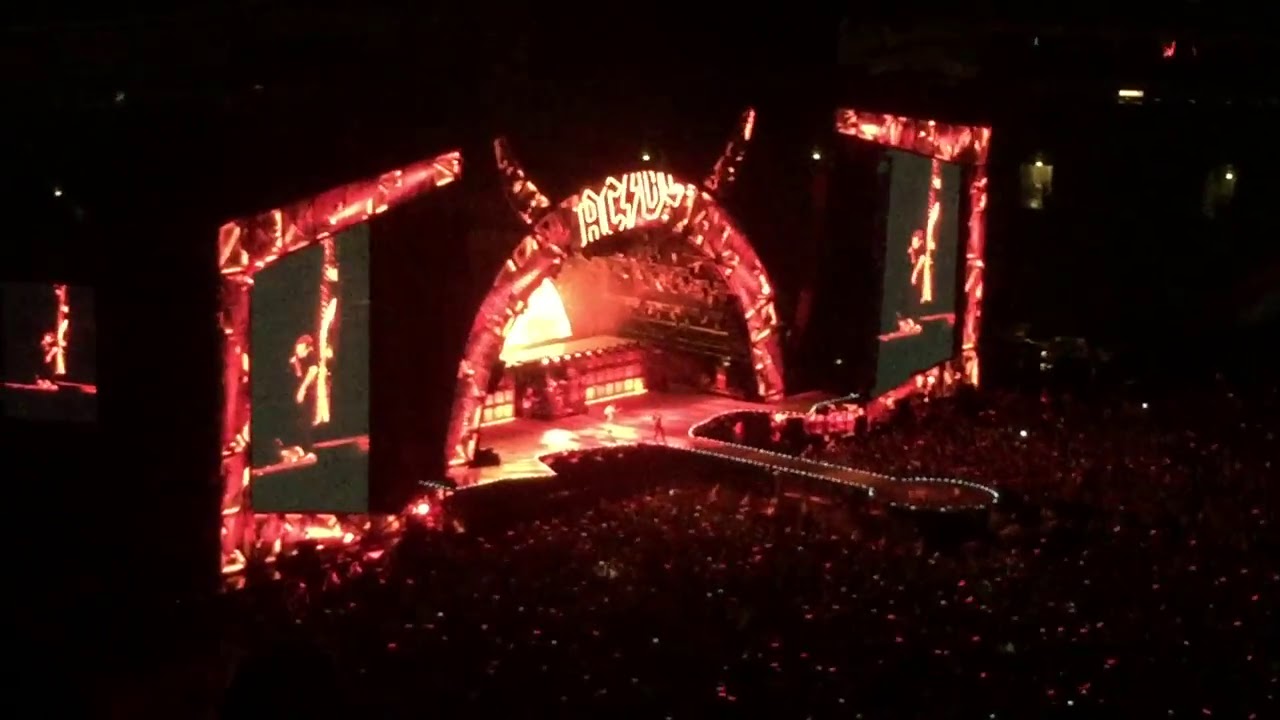This high-angled, nighttime photograph captures a dynamic rock concert, presumably one by AC/DC, taking place on an intricately designed, well-lit stage. The stage is framed with fiery red and orange lights, giving it an intense glow. At its center is a prominent arch with the iconic band's name, “AC/DC,” featuring their lightning bolt logo, flanked by devil horns on top. Surrounding the stage are large, rectangular panels also trimmed in red, enhancing the fiery motif. A lit runway extends from the stage into the audience, ending in a circular platform.

The photograph showcases a throng of concertgoers densely packed in front of the stage, their silhouettes illuminated sporadically by the stage lights. Two large screens on either side of the stage display the lead performer, whose indistinguishable figure raises hands, likely engaging with the crowd. The reddish-orangish glow dominates the center stage, contrasting sharply with the surrounding darkness filled with scattered lights from the audience. The overall scene conveys the electrifying atmosphere of a live rock concert, with the audience energy palpable even in still imagery.